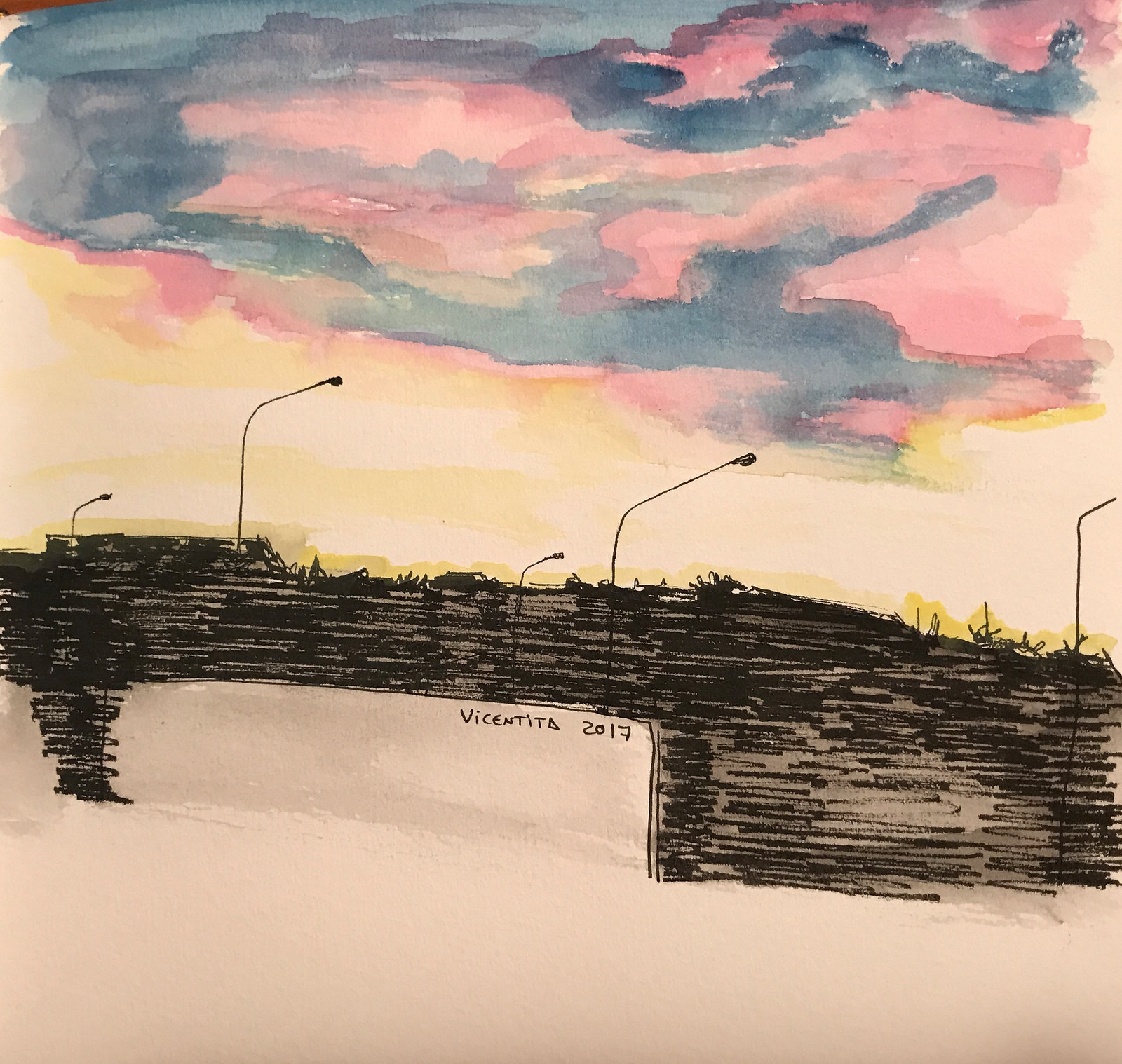This detailed artwork, titled "Vicentita 2017," appears to be a harmonious blend of watercolor and ink on off-white, square paper. The sky, likely depicting a sunset, showcases a stunning palette of blues, pinks, grays, and yellows, with colors streaking through cloud formations. Below the vibrant sky, a prominent black structure, resembling a bridge, stretches horizontally across the composition. The bridge is meticulously detailed with horizontal scribbled lines in black ink or marker, evoking its textured surface. Tall, slender streetlights with small, round bulbs angle gracefully over the bridge, adding a delicate touch to the scene. At the base of this intricate artwork, the bridge forms a sharp 90-degree angle, under which the artist's signature, "Vicentita 2017," is finely inscribed in black. The lower section of the piece remains stark white, providing a striking contrast to the colorful sky above.